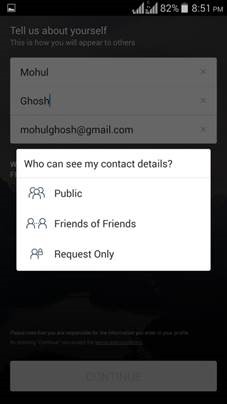The image depicts a smartphone screenshot of a website interface. The primary screen has a black background with some text partially obscured by a prominent pop-up window. The pop-up window has a white background with dark gray or black text. The header of the pop-up reads, "Who can see my contact details?" followed by a question mark.

Below this header, the pop-up displays three options, each accompanied by an icon:
1. **Public**: Illustrated with a generic avatar.
2. **Friends of Friends**: Shown with two user icons connected by a line.
3. **Request Only**: Represented with a single user icon and another person icon in the background.

This pop-up overlaps the underlying page, indicating it is an active dialogue box requiring user interaction. 

At the top of the screen, the status bar displays a Wi-Fi signal icon, an 82% battery charge, and the current time, 8:51 PM.

The content beneath the pop-up is partially visible and appears to be a profile input form with the heading, "Tell us about yourself. This is how you will appear to others." The form includes fields pre-filled with:
- **First Name**: "Mohul" (all uppercase)
- **Last Name**: "Ghosh" (all uppercase, though misspelled in transcription it should be "Ghosh")
- **Email Address**: "mohulghosh@gmail.com"

To the right of each field, there is an "X" icon, presumably for clearing the entered information. At the bottom of the screen, a banner with the text "Continue" signals the next step in the process.